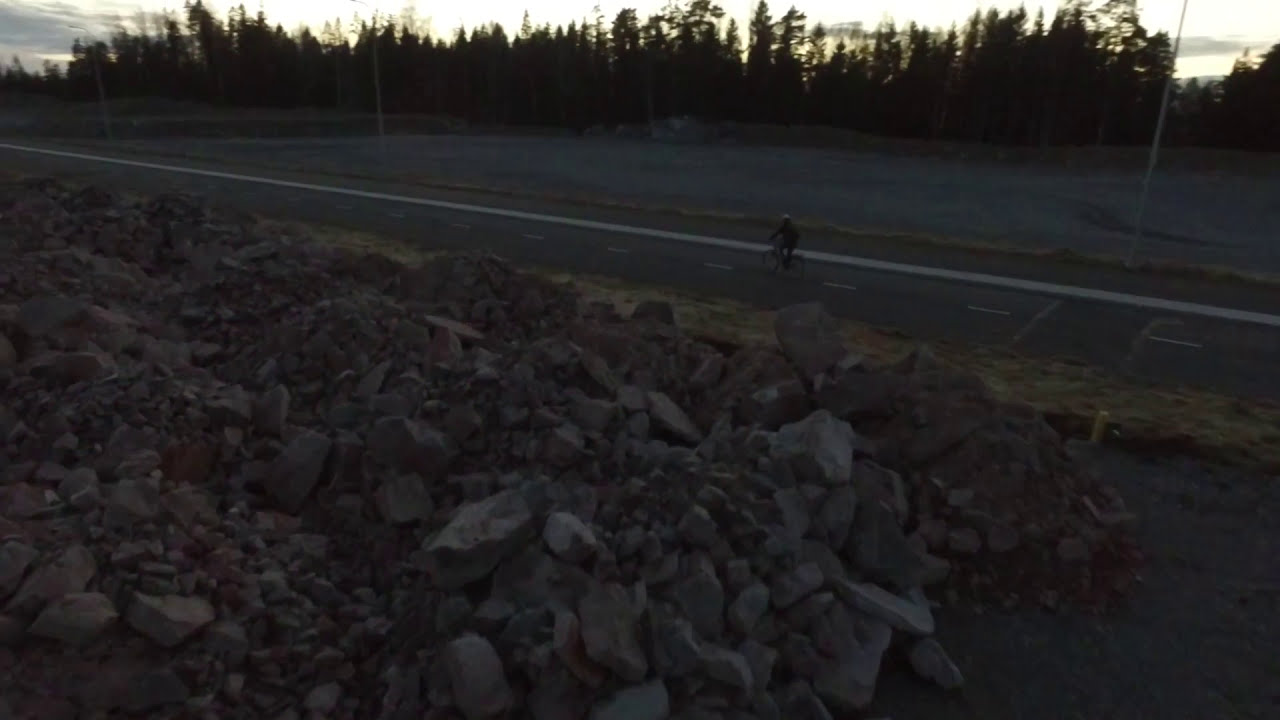The image captures a dusky, outdoor scene featuring a lone bicyclist riding along a one-lane road marked with white lines. The setting is characterized by a prominent pile of gray and darker rocks in the foreground, occupying nearly half of the image. Above the rock pile lies the road, stretching horizontally across the scene with the cyclist, helmet visible, traveling towards the left. The overall lighting suggests evening or early night, as the sky remains faintly illuminated by the sun that has already set, casting a glow despite the presence of gray clouds. The backdrop includes a tree line silhouetted in black against the sky, further contributing to the low-light ambiance. The scene is devoid of any text or additional human presence, emphasizing the solitude of the cyclist amidst the natural and rugged terrain.